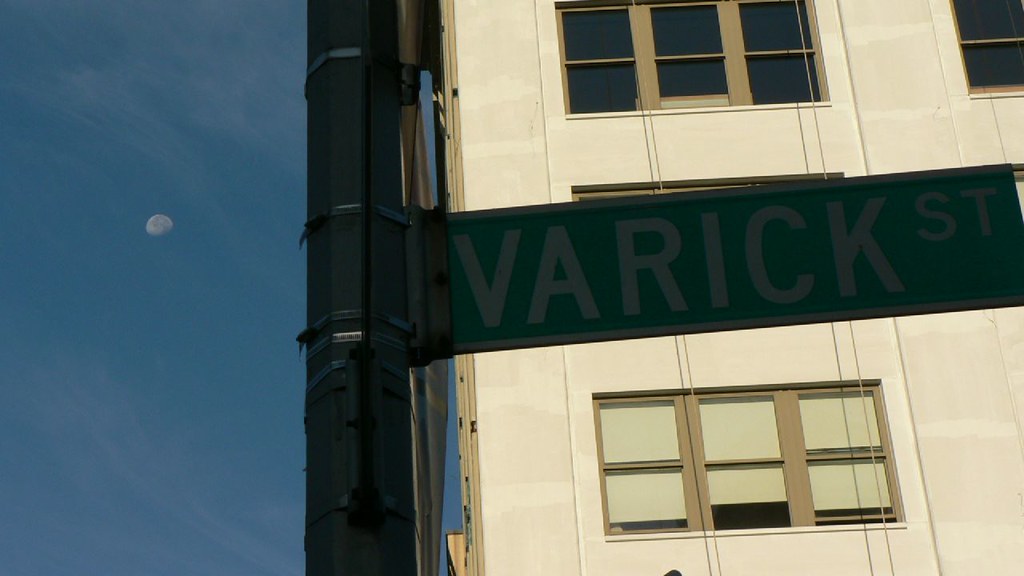In the foreground of the image, a street sign reading "Varick Street" prominently faces the camera. The sign is colored green with white letters and outlines, typical of street signs in an American city. It is affixed to a tall, black pole, although the full length of the pole is not visible due to the zoomed-in nature of the photograph. The background features a large building, which occupies more than half of the image, casting a shadow that partially darkens the sign. In the upper left corner of the image, a pale moon hangs in the sky, adding an ethereal touch to the urban scene.